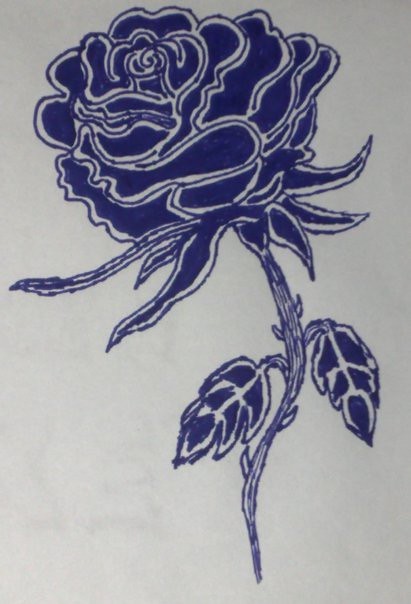The image is a photograph of a detailed sketch or painting on white paper, predominantly executed in blue pen or marker. It showcases a beautifully detailed, fully bloomed rose with numerous petals gradient from larger ones at the bottom to smaller ones towards the center. The petals are outlined in white, with a finer blue trim between the white and the deep blue shading, giving the rose a multi-dimensional effect. Starting from the top middle of the image, the flower head leans slightly to the left. Beneath the rose, there are six slender, pointed leaves arranged around the base of the flower, all outlined in white and filled with blue shading. The stem, depicted with a slight curve, extends downward and features a couple of small thorns along with two leaves, one on each side, similarly styled with white outlines and blue shading. The overall image has no textual elements or signatures and appears to shift slightly in color due to the photo's exposure, possibly giving the white background a faint grayish hue.